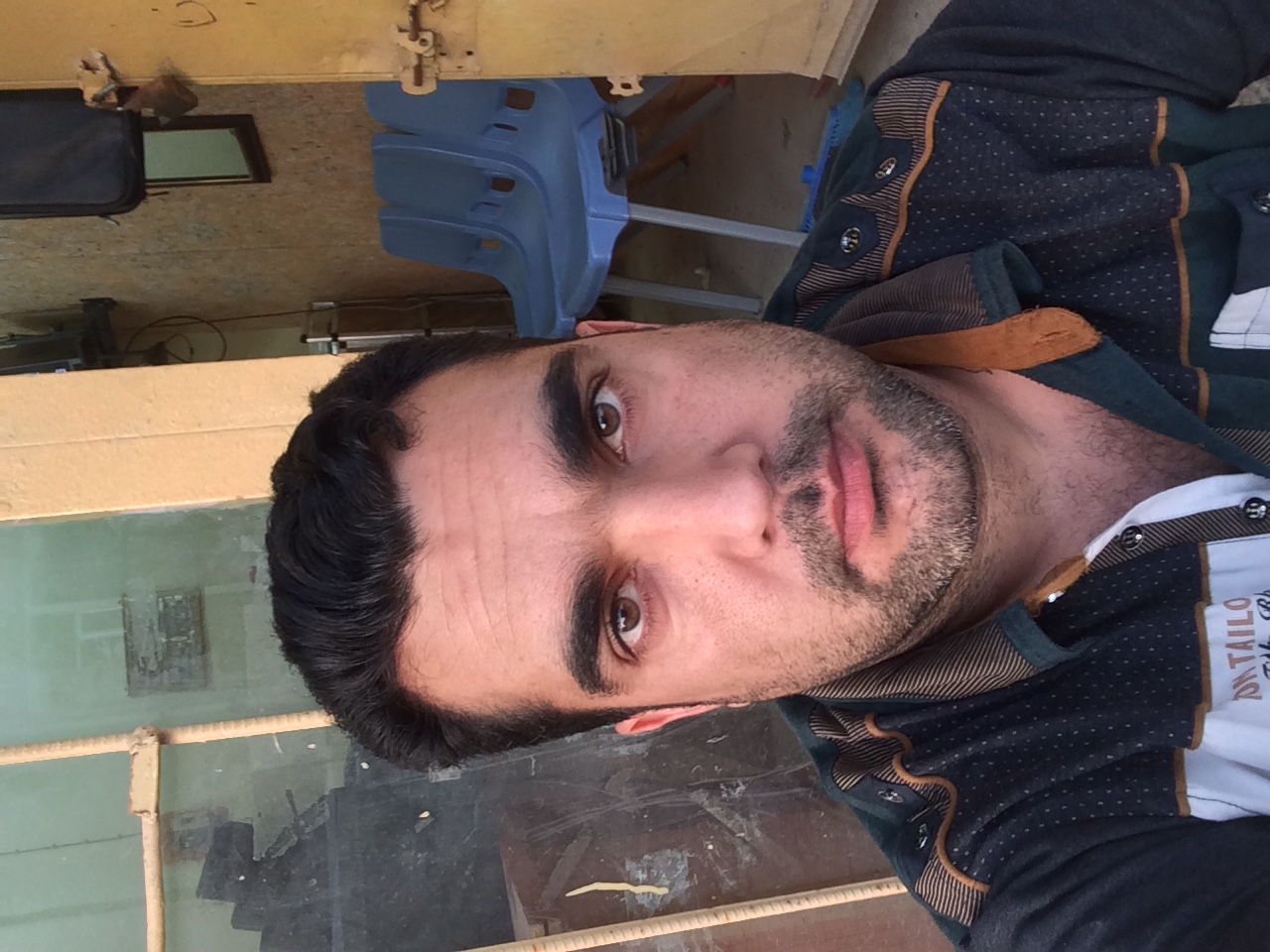This is a selfie of a Hispanic man with tan skin, large bushy black eyebrows, dark brown eyes, and a black five o'clock shadow complemented by a goatee. His dark black hair is of medium length, typical for a man. He gazes directly at the camera, wearing a distinctive button-up collared shirt that is black with polka dots. The shirt is unique, featuring buttons on the shoulders and an obscured white stripe with the letters "o-n-t-a-i-l-o." The background gives a glimpse into a somewhat rustic and secure setting, with three blue chairs lined up against a plywood wall and a door outfitted with multiple locks. An outbuilding, painted light tan with rebar visible on the exterior, has a window through which a mirror is visible, adding to the intriguing details of the scene. The lighting and setting create ambiguity about whether the photo was taken during the day or night and whether it was indoors or outdoors.